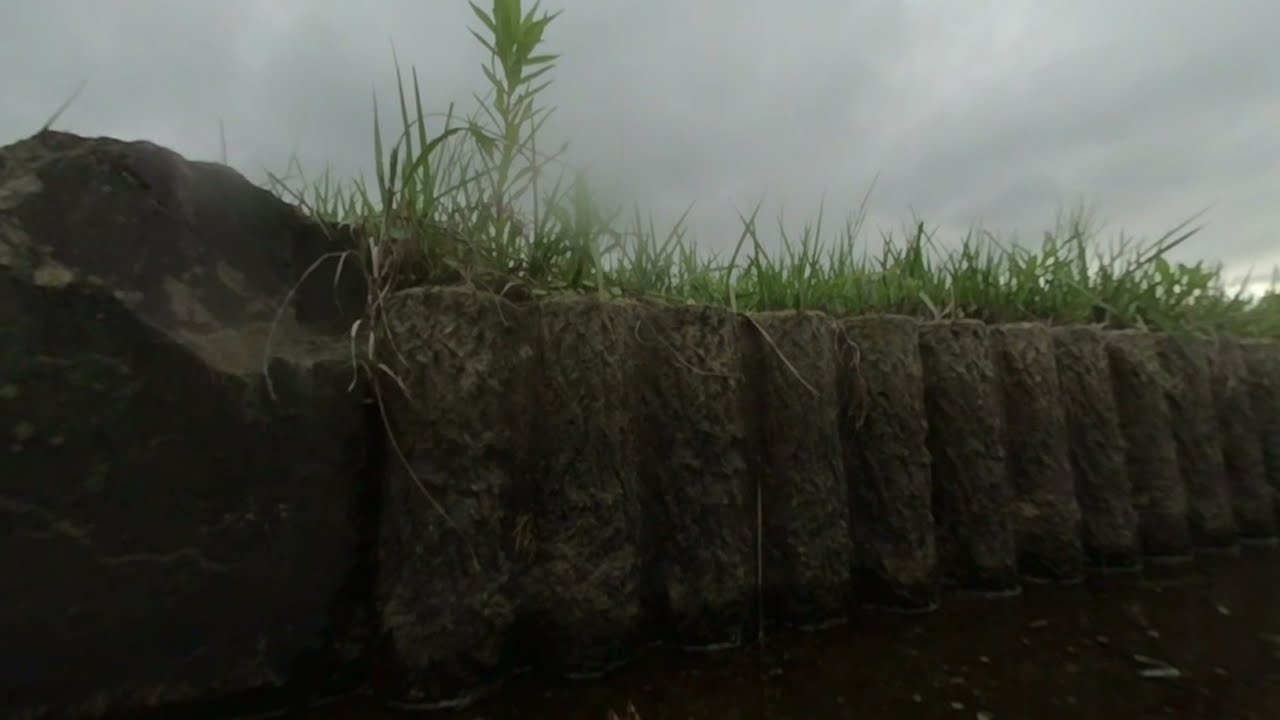The image depicts an outdoor scene with a very gray and cloudy sky, indicating an overcast day that looks like it might rain. Dominating the lower half of the image is a pattern resembling a garden edge or barrier formed by cylindrical, tubular posts lined up vertically. These symmetrical pillars are brown and appear to be made of dirt, wood, or a similar material, and stretch from the middle to the right side of the image. The foreground is quite dark, casting shadows that make it challenging to discern specific details. To the left, there is a rocky area that protrudes upwards slightly. Behind and possibly on top of these tubular posts, lush green grass and various plants and weeds grow. In the far right corner of the upper half, there is a faint hint of daylight peeking through the dense cloud cover. Overall, the scene has a somber and stormy atmosphere, with no visible sun or text elements anywhere in the picture.